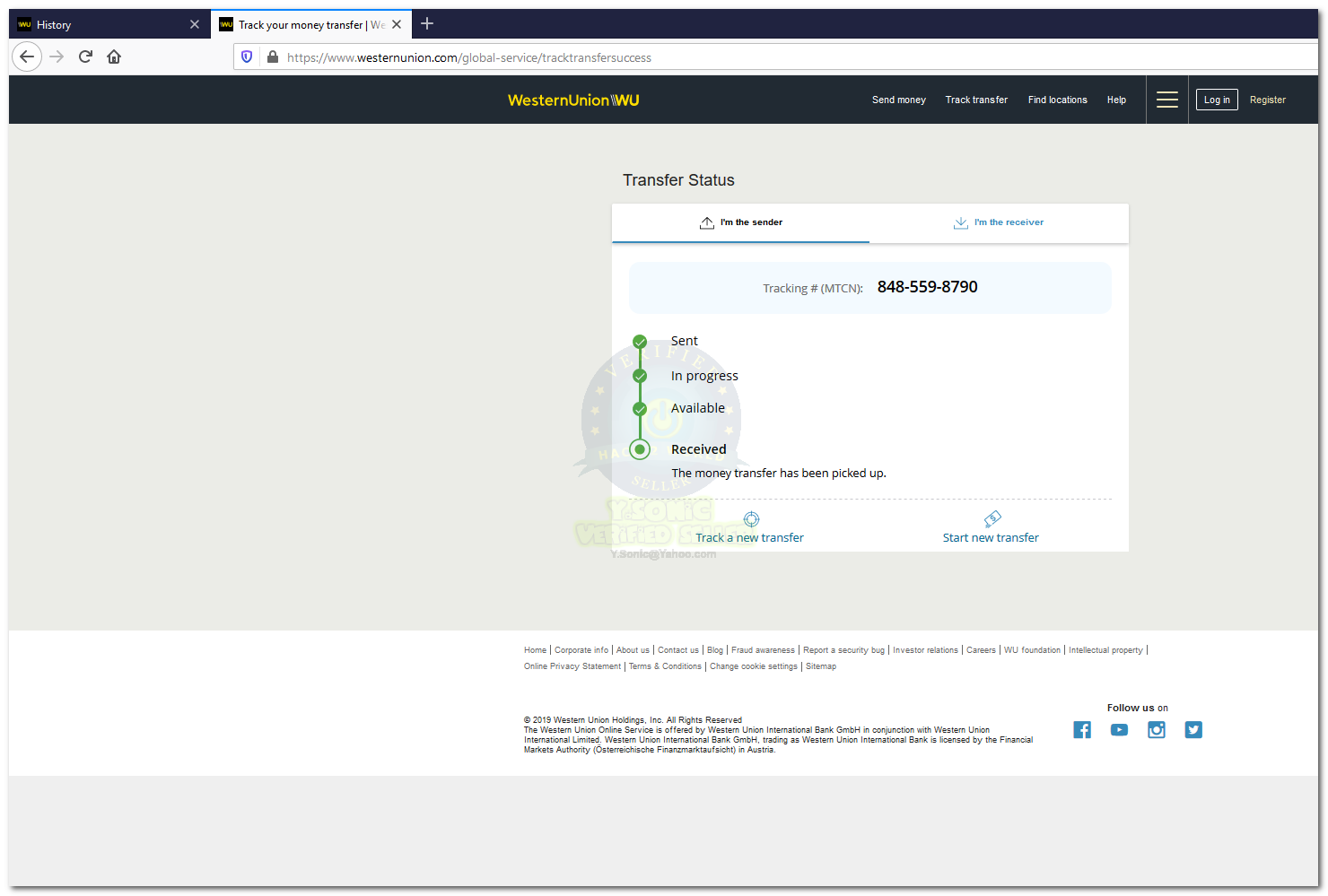Screenshot of a computer screen displaying the Western Union money transfer tracking page.

The browser's tabs at the top indicate the current page as "Track Your Money Transfer", with a second tab labeled "History". The URL displayed is "westernunion.com/global-service/track-transfer-success", signaling a successful transaction tracking page from Western Union.

In the main section, a pop-up box is visible featuring options for "I'm the sender" or "I'm the receiver," with "I'm the sender" selected. The tracking number (MTCN) provided is 848-559-8790.

A vertical progress indicator on the left side highlights the stages of the transaction:
- "Sent" - Marked with a green checkmark.
- "In Progress" - Marked with a green checkmark.
- "Available" - Marked with a green checkmark.
- "Received" - Indicated by a green circle.

A notification confirms that the money transfer has been picked up.

At the bottom of the page, there are links to "Home," "Contact Us," and "About Us," along with icons prompting users to follow Western Union on Facebook, YouTube, Instagram, and Twitter.